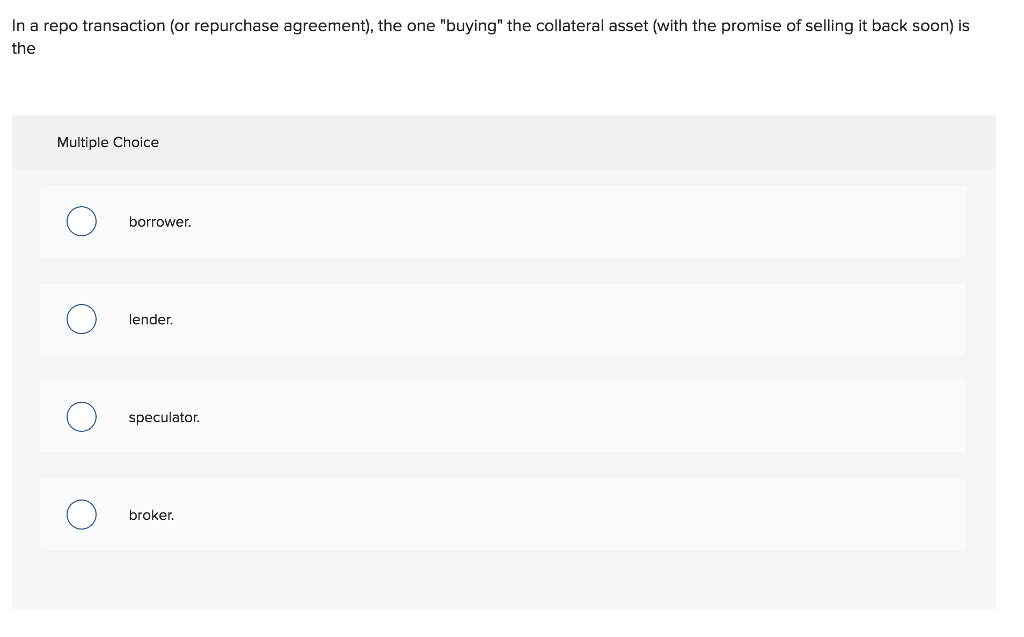The image features a multiple-choice question prominently displayed on a white background. At the top, in black text, is the question: "In a repo transaction (or repurchase agreement), the entity 'buying' the collateral asset (with the promise of selling it back soon) is the __." Below this question is a gray box labeled "Multiple Choice," containing four possible answers in a slightly lighter gray box. Each option is prefaced by a blue circle and is written in black text. The choices are as follows: 

1. Borrower.
2. Lender.
3. Speculator.
4. Broker.

The design presents a clear contrast between the white background, the gray boxes, and the black text, ensuring the question and answer choices are easy to read. There are no other elements present on the screen.